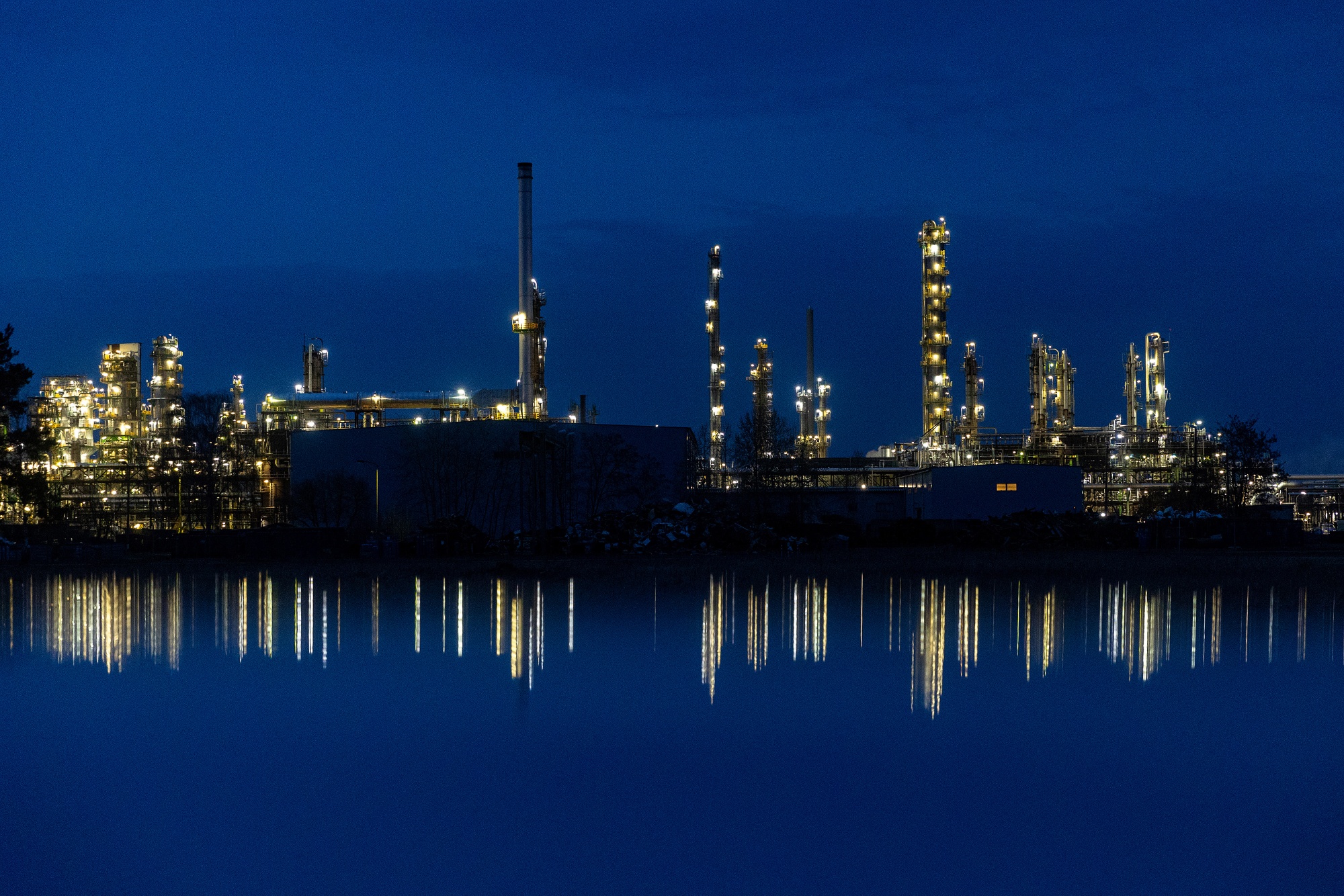This photograph captures a mesmerizing nighttime city skyline, predominantly illuminated by whitish-yellow lights that paint the scene with a luminous glow. Standing beside a dark navy waterfront, the city's reflection in the water creates a striking mirror image. The skyline comprises various tall buildings, smokestacks, and industrial towers, suggesting the presence of an oil refinery or similar industrial site. Central to this image is a factory smokestack on the left and several other towers stretching into the night sky. On the left edge of the photo, a tree pokes into view, complemented by another more distant tree on the right. In front of the waterfront, a line of grass separates the water from urban structures, including a prominent large building and a smaller one with a single lit window, possibly a residential area. Although the industrial elements may not be inherently beautiful, the photo transforms the scene into a captivating panorama by the serene, dark blue sky and its flawless reflection on the water below.